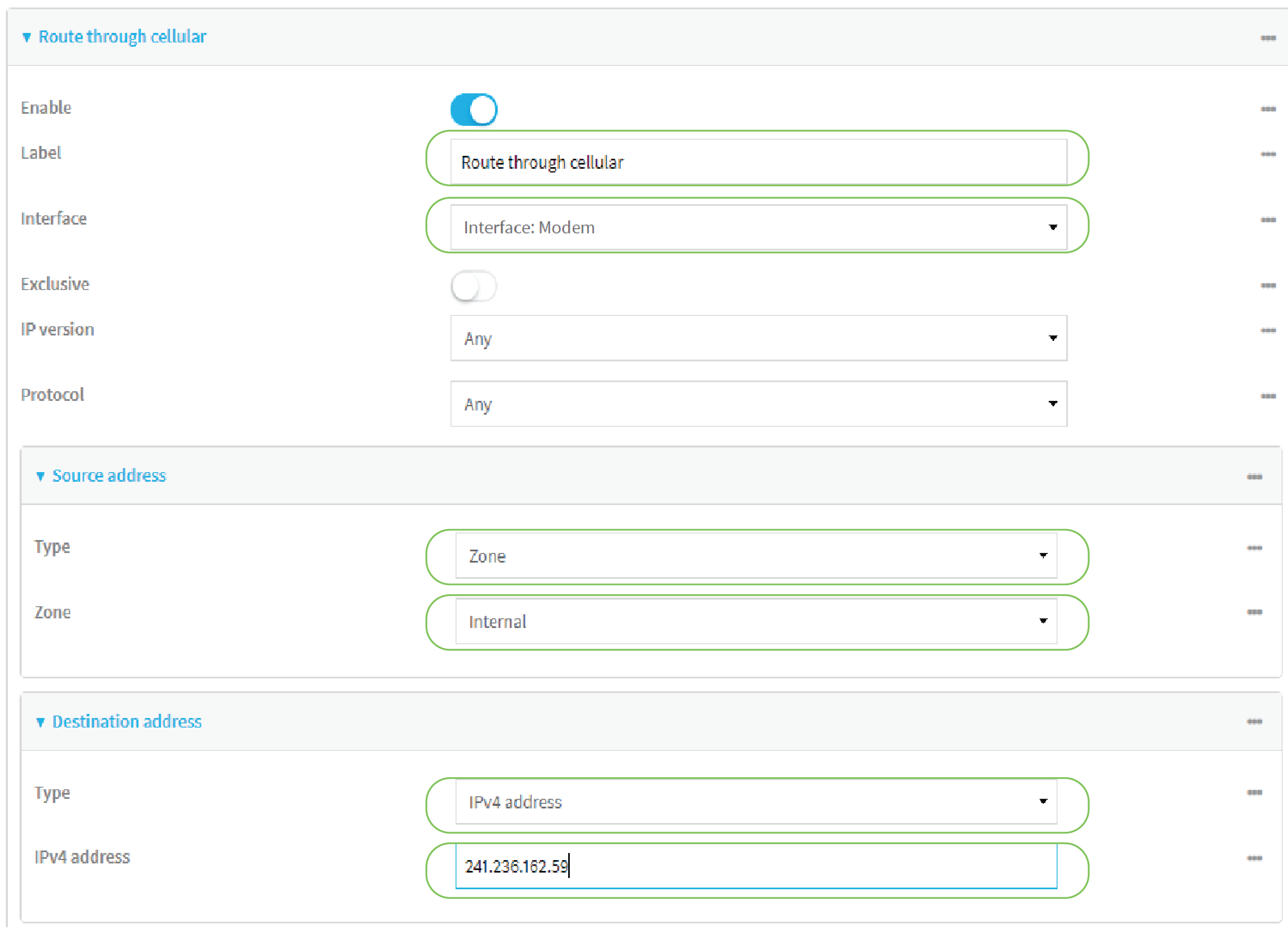The image displays the settings interface of a router, specifically focused on routing through a cellular connection. 

At the top, the interface has a section labeled "Route through cellular" written in blue letters, accompanied by a blue drop-down arrow. Below this label, it states "Enable" in black letters, which is activated using a blue toggle button.

Following that, there's a section labeled "Label" with a green circular border surrounding a box that again contains the text "Route through cellular."

Next, the interface outlines several settings: 

1. **Interface**: Displays "Modem" within a green-circled box.
2. **Exclusive**: This option is turned off.
3. **IP Version & Protocol**: Both set to “Any” and enclosed in a square box with a drop-down arrow.

Further down, the settings for **Source Address** appear in blue letters with an accompanying drop-down arrow. This section includes:

- **Type**: Listed as "Zone" within a square box that has a green circular border.
- **Zone**: "Internal" is the selected option, also enclosed in a square box with a green border and drop-down arrow for altering these settings.

Lastly, at the bottom of the interface, the **Destination Address** is specified in blue letters with a blue drop-down arrow. This includes options for:

- **Type**: Set to "IPv4 Address" within a box bordered by a green circle.
- **IPv4 Address**: Displays the IP address "241.236.162.59" inside a similarly bordered box.

This detailed setup helps configure precise routing rules for cellular connections on the router.